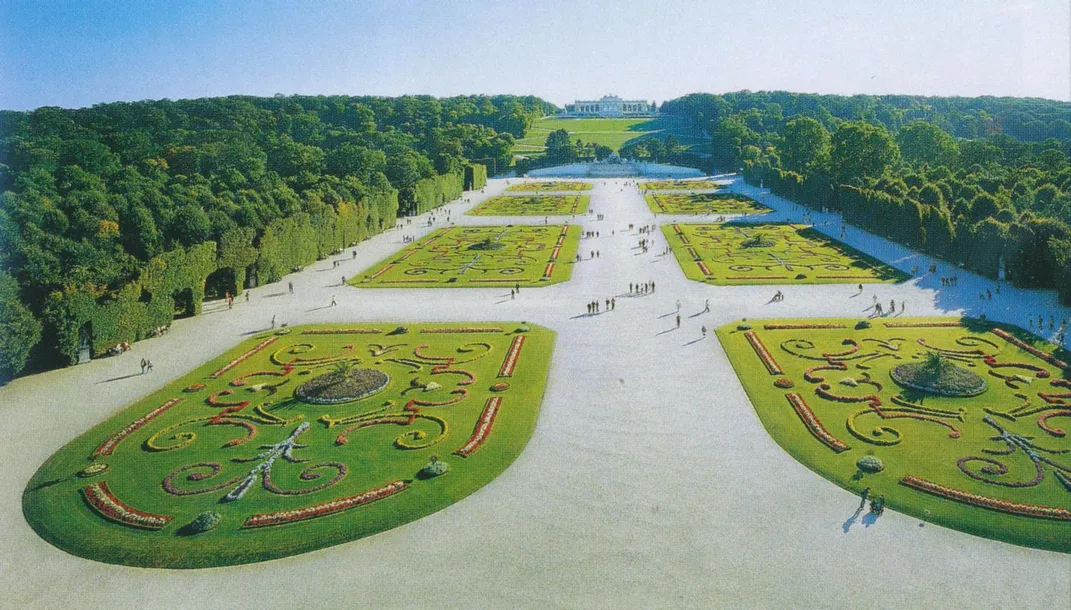This digital artwork depicts a sprawling field, meticulously segmented with geometric patches of carefully trimmed grass and intricate floral designs. The vast expanse is bordered by tall, precisely manicured trees, lending an artistic and somewhat surreal aspect to the scene. Scattered throughout the field are numerous figures, adding a touch of humanity to the otherwise stylized environment. In the background, perched on a hill, stands a grand mansion with stately columns, offering a focal point amidst the sea of greenery. The blend of nature and man-made elements, along with the precise detailing of the landscape, underscores the creator's technical proficiency and imaginative vision.